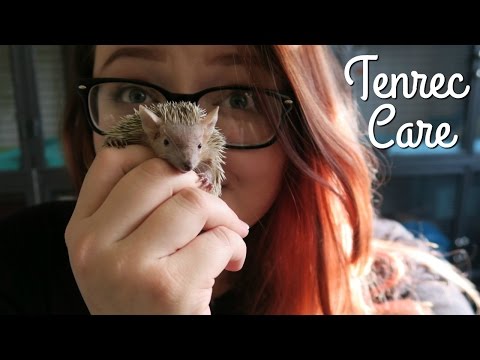In the image, an overweight Caucasian woman in her mid to late 20s, possibly appearing older due to her presentation, holds a small, spiky beige hedgehog over her nose and mouth. The hedgehog’s beady black eyes and brownish face peek over her fingers. Her hand obscures much of her facial expression, but her raised eyebrows behind her thick black-rimmed glasses suggest she is happy. She has dark red, slightly wavy hair illuminated by natural sunlight, hinting at an indoor setting with a window partially visible on the left side. The picture features the text "Tenrec Care" in white, cursive font on the right side, indicating it may be the thumbnail for a video on hedgehog care. The photo is bordered by solid black horizontal lines at the top and bottom.